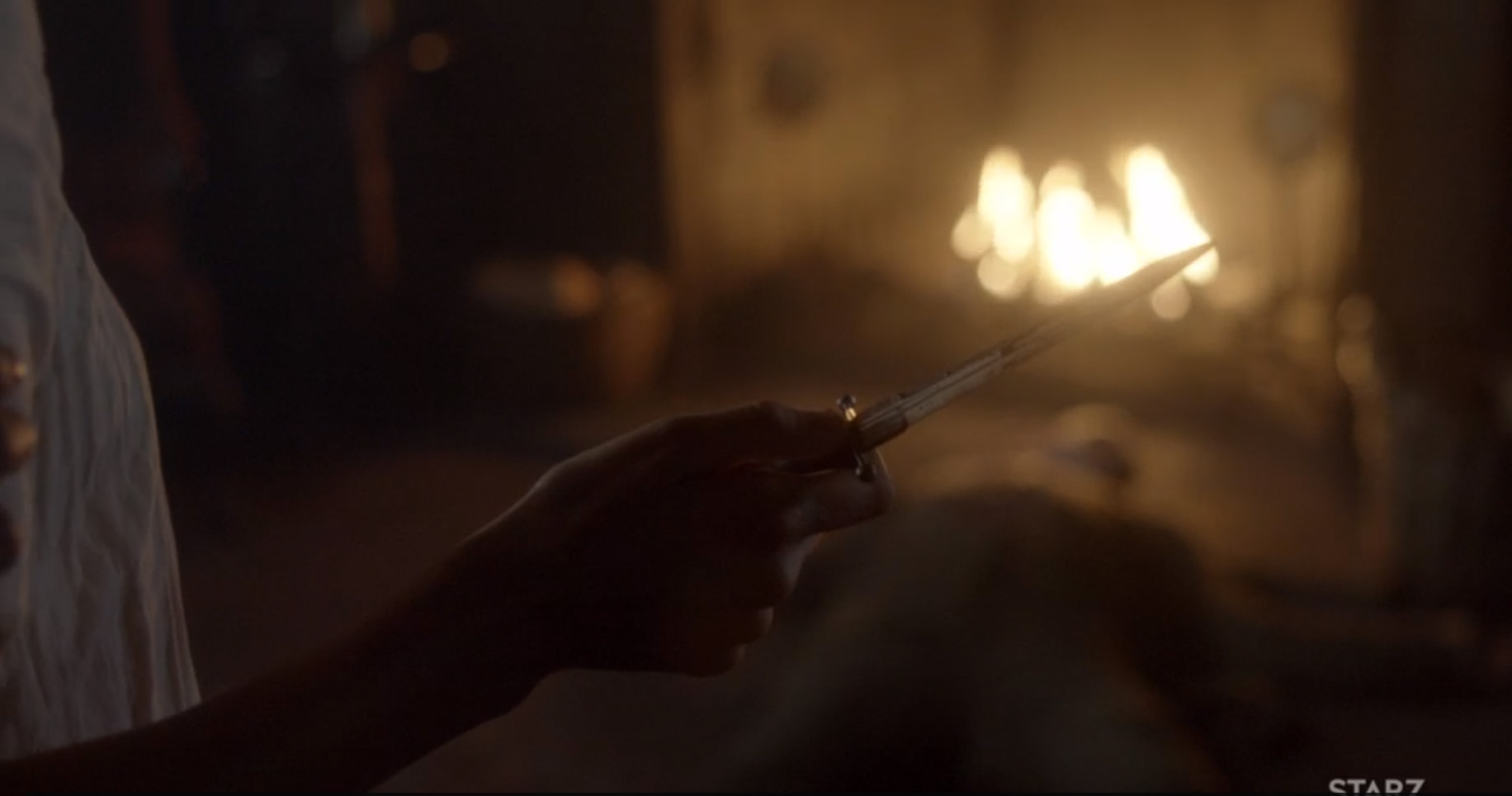The image appears to be a screenshot from a television show, identifiable by the "STARZ" watermark located in the bottom right-hand corner. The scene is dimly lit, with a blurred background dominated by what seems to be a fireplace, casting a warm, flickering light throughout the space. 

In the foreground, a person, presumably a woman, stands holding a knife or a similarly sharp object. Due to the intensity of the backlighting from the fire, discerning specific details such as skin color is challenging, though it might be brown. The woman appears to be dressed in a white outfit or gown, which contrasts sharply against the darker, shadowy surroundings. The overall mood of the image is suspenseful and mysterious, enhanced by the dim and blurred ambiance.